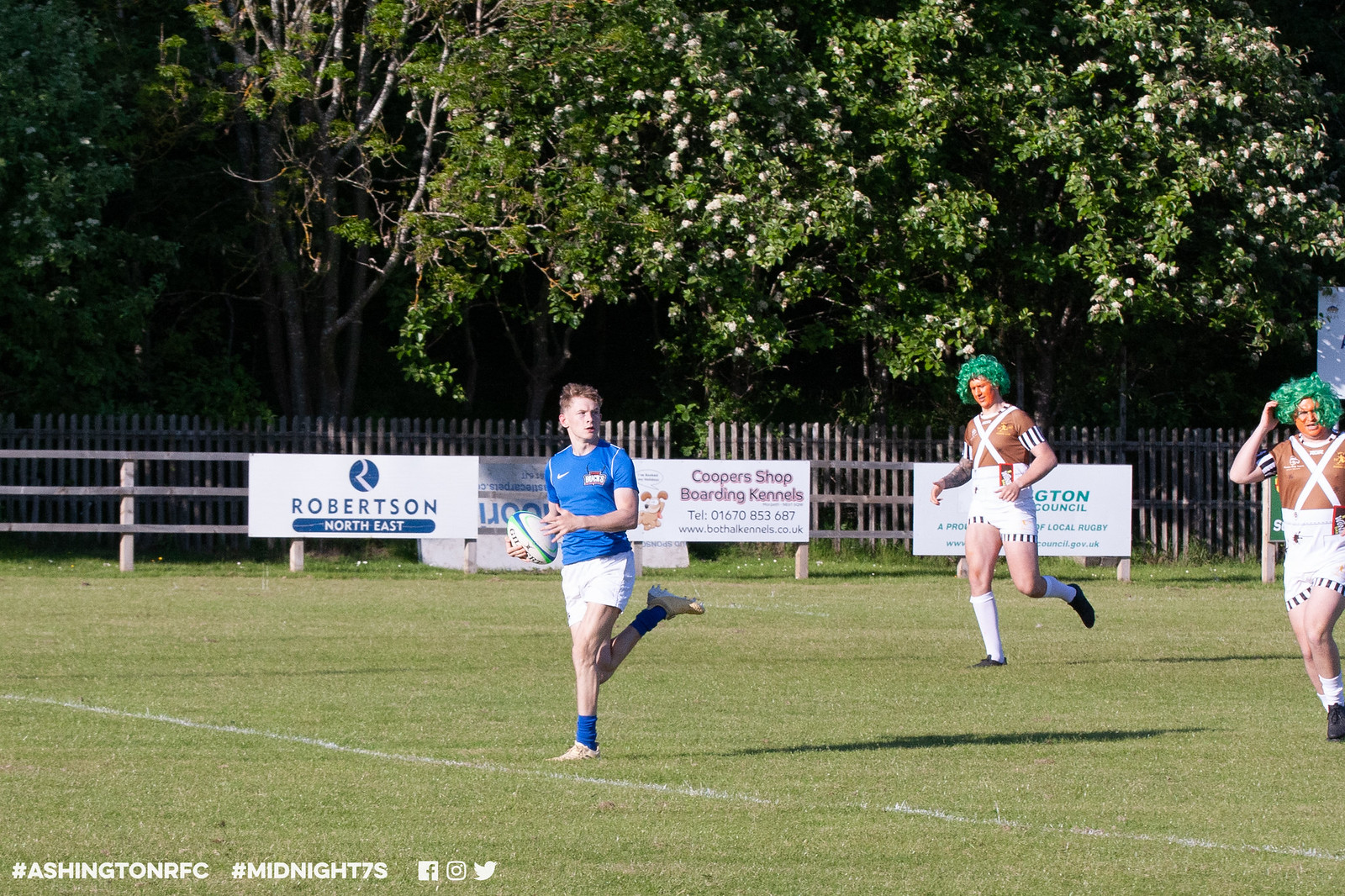This outdoor scene captures a lively moment on a grassy field where three men are engaged in an activity reminiscent of a college event. At the center of the image, slightly to the left, stands a man wearing a blue shirt, white shorts, and blue socks. Behind him, two men can be seen running in the same direction, sporting quirky green wigs, brown shirts, white shorts, and black shoes, with their faces painted brown. Interestingly, they appear to be wearing costumes resembling lederhosen, but the suspenders are worn backwards.

The field is enclosed by a fence adorned with various advertisements. Among them, one sign prominently displays "Robertson Northeast," while another reads "Cooper's Shop Boarding Kennels," featuring an image of a dog and a phone number 016-708-53687. At the bottom left corner of the image, "Ashington RFC" and "Midnight 7s" are hashtagged alongside social media icons for Facebook, Instagram, and Twitter.

In the background, large bushes with white blossoms stand tall, almost tree-like, adding a natural border to the scene. The field itself is marked with white lines, enhancing the impression of an organized sporting event.